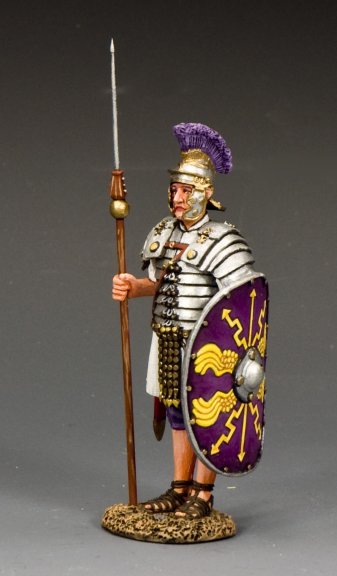The image showcases an action figure of a Roman legionary soldier standing against a grayish background. The soldier, a male figurine, is dressed in segmented plate armor with intricate layers of silver and gold, and a leather strap crossing over the front. He wears traditional Roman leather sandals with mini straps on his feet. His head is adorned with a striking gold and silver helmet, featuring a large purple plume running like a mohawk along the top.

In his right hand, the figure holds a long spear with a thin tip and a small golden ball connecting the metal head to the wooden shaft. His left arm is equipped with a large, ornate shield that covers half his body. The shield has a purple base with decorative gold designs, including yellow arrows and tassels, and a central silver steel circle.

The soldier appears to be standing on a yellow and black spotted rock, serving as a base to prevent the figure from toppling over. The attention to detail in the craftsmanship, from the plated armor and segmented skirts to the elaborate shield and distinctive helmet, highlights the historical accuracy and artistic quality of the figurine.